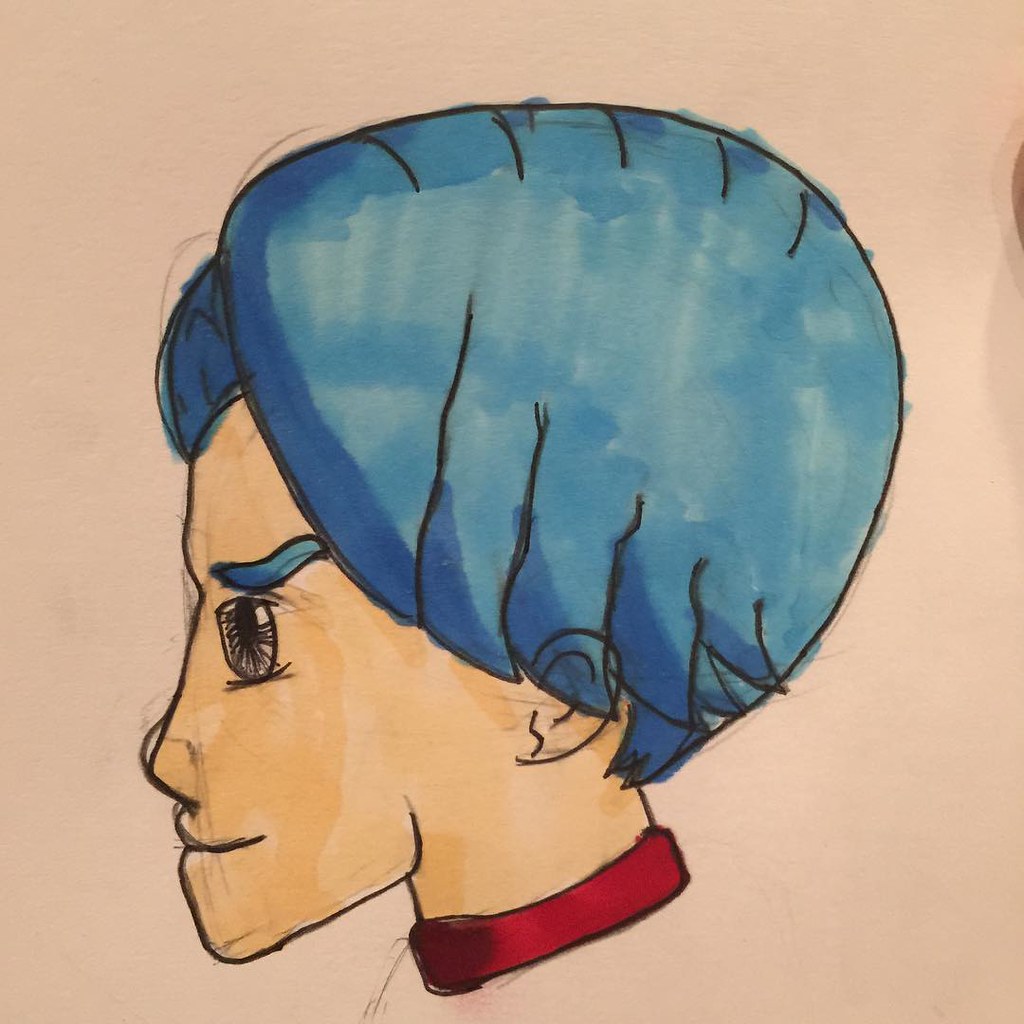This is an expressive illustration of a girl's side profile adorned with short blue hair, rendered with what appears to be markers and possibly watercolors. The hairstyle slightly extends past her ears, with the blue hue intensifying towards the tips, creating a wet paper effect where the marker saturates heavily. Her hair, eyebrows, and a prominent eye are vividly blue, with the eye encircled by simplistic black lines. The girl's other facial features include a small, slightly upturned nose, and lips that appear pursed. She wears a distinct red necklace or collar. The background of this piece is a pink to off-white, peachy tone, with some blue coloring lapsing outside the black outline of her head. This side profile captures her with a light, peachy skin tone, and a poised look directed towards the left, painted on a somewhat textured paper.